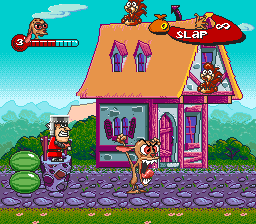In this detailed screen capture from a Ren and Stimpy video game, the scene is vibrant and packed with quirky elements. In the foreground, Ren, who is light tan with an oversized head and a very expressive, raging face—his mouth open, jagged teeth exposed, and eyes bulging red—is standing on a cobblestone road depicted in alternating dark blue and light blue stones. His fists are clenched, and he appears animatedly angry, looking towards the right. A simple green grass strip, dotted with subtle white and black flowers, lines the immediate foreground.

Behind Ren, to the right, stands a whimsical one-story house with distinct blue walls, pink trim, and a light yellow roof. The house features two small windows on its sides and one at the front, near a vividly pink door flanked by pink columns. On the roof, several squirrels scurry about near a banner adorned with the word "SLIP" in white lettering.

To the left of Ren, a blue and brown stone well harbors a small man emerging from it, dressed in a red jacket. Further to the left, in the far corner, two green watermelons with darker green stripes are neatly stacked on top of each other. The sky above is a light teal, and in the upper left corner of the image is an overlay resembling a horizontal thermometer with a chihuahua or similar character appearing from it. The overall aesthetic is reminiscent of a retro, colorful platformer video game.